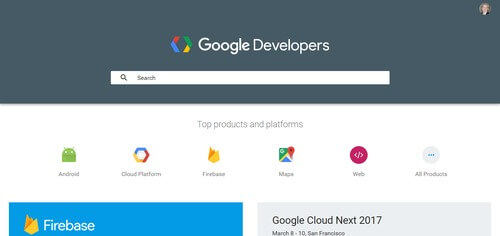The image showcases a section of the Google Developers webpage. At the top, the words "Google Developers" are prominently displayed, followed by a search bar situated directly beneath it. The central portion of the image features a list of top products and platforms, including Android, Cloud Platform, Firebase, Google Maps, and Web, with an additional link to view all products. 

A highlighted section mentions "Firebase" along with an event: "Google Cloud Next 2017," which is scheduled to take place from March 8 to 10 in San Francisco. 

In the top-right corner, there is a digital photograph of the user. The overall color scheme of the webpage encompasses shades of green, orange, yellow, blue, gray, and white, lending the interface a vibrant yet professional appearance.